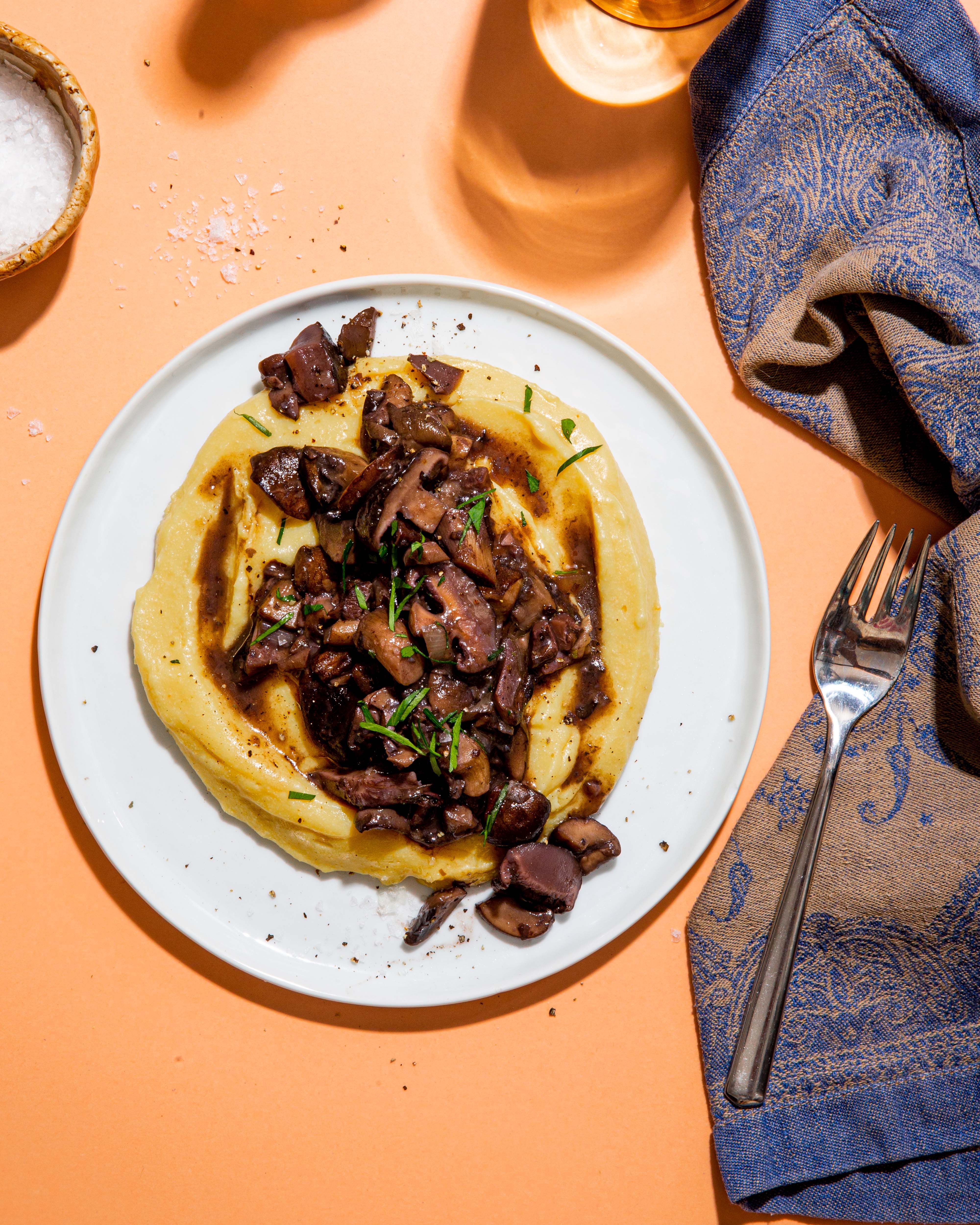This top-down color photograph captures a rectangular image showcasing a meticulously arranged plate of food at its center. The centerpiece is a white, shallow, porcelain plate featuring a circular mound of mashed potatoes generously topped with tender beef tips and a rich, dark brown gravy. Scattered over the meat are fresh green herbs, possibly cilantro, adding a vibrant touch of color. This entire ensemble sits on an orange table. To the right of the plate lies a four-pronged fork placed neatly atop a blue and brown napkin. In the top left corner of the image, a small wicker basket of salt is subtly included. The careful composition emphasizes the savory appeal and inviting presentation of the dish.